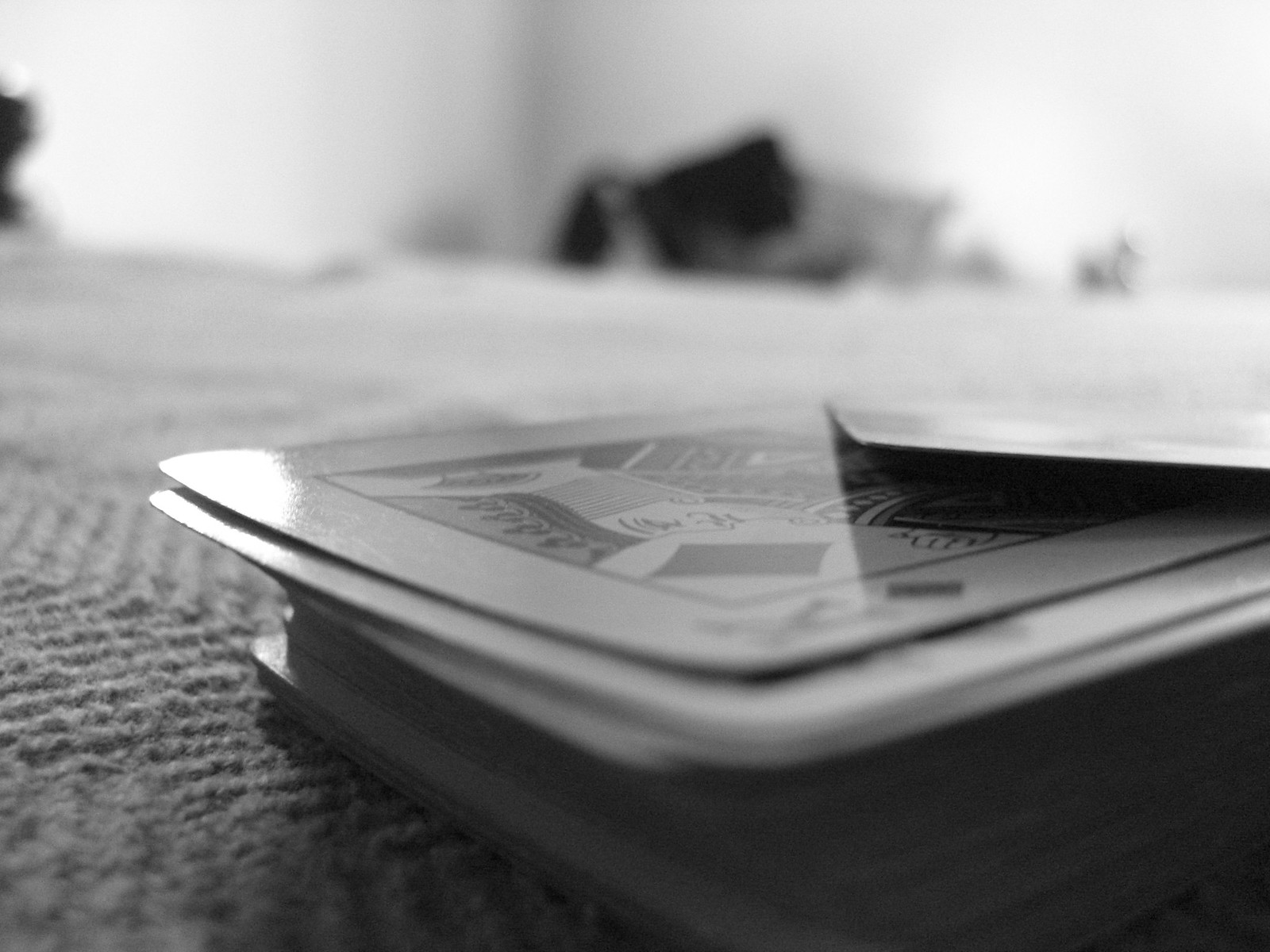Close-up Black and White Image Featuring an Ambiguous Scene: The photo is a blurred, monochromatic capture, making details hard to discern. In the background, faint outlines of two windows can be seen, draped with sheer, opaque white curtains against a white wall. Between the windows, there appears to be an indistinct pile of objects, presenting varying shades of light and dark, contributing to the scene's mystery. In the foreground, likely on a table with a woven mat, there is a stack of thick cards. The cards are splayed slightly to the left, with one card notably separated to the right. Although the specific type is unclear, they appear to resemble tarot cards due to their thickness and partially visible illustrations, including a rectangle and a possible face.